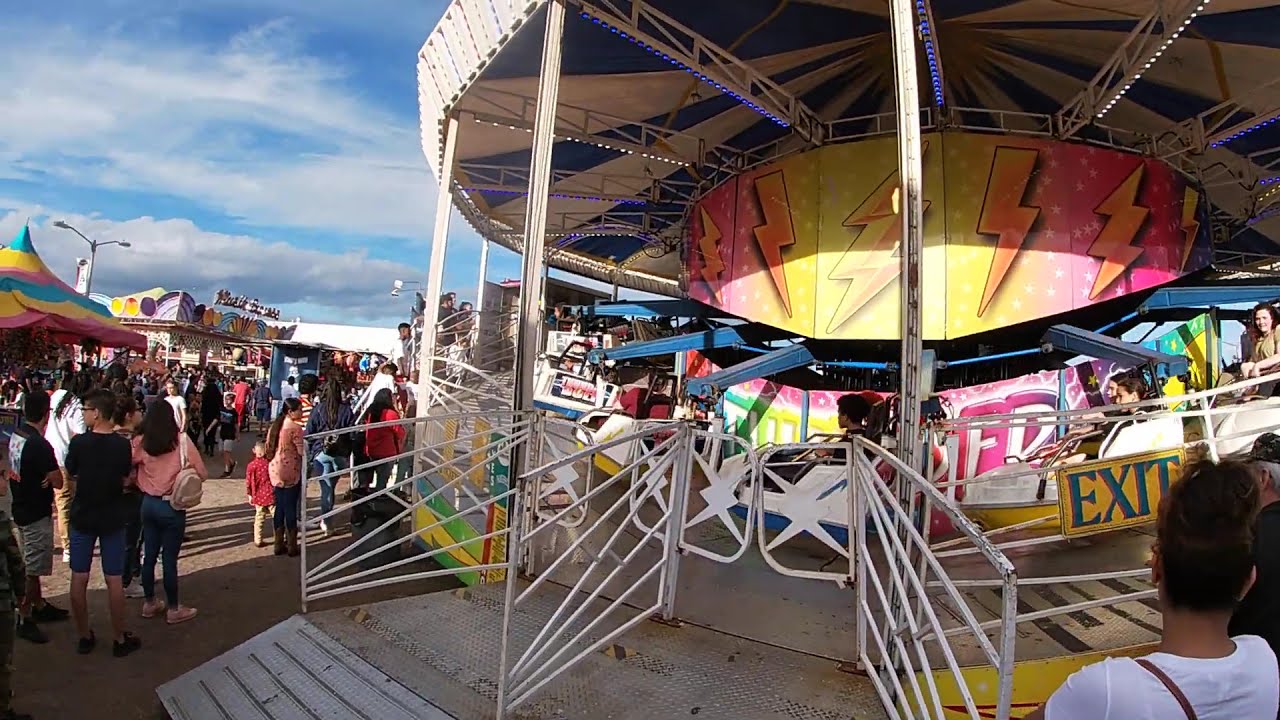The image depicts a vibrant, outdoor carnival scene set on a stone or concrete ground surface and taking place in the middle of the day. Dominating the center of the image is a large, colorful carousel with seats that rotate and move up and down. The carousel features a striking color palette with a white top adorned with purple and white LED lights, orange lightning bolts on a pink, yellow, and orange backdrop, and white stars painted around it. Blue arms extend out, holding seats occupied by multiple passengers, and a gate surrounds the ride, indicating a yellow exit sign with more people standing in line.

To the left of the image, there is a bustling crowd of dozens, if not hundreds, of carnival-goers. Among them is a woman in a pink shirt, blue jeans, and with a purse over her shoulder. The area features various food stands and tents, including a large tent with a blue, yellow, and pink canopy and an open building with a similarly colorful roof. Despite some writing on the structure, it remains indistinct. A streetlamp can also be seen above this area.

The sky above is a light blue with sparse white clouds, adding to the cheerful ambiance of the carnival. The entire scene bursts with vivid colors such as light blue, white, gray, yellow, pink, turquoise, orange, and silver, encapsulating the lively spirit of the carnival.